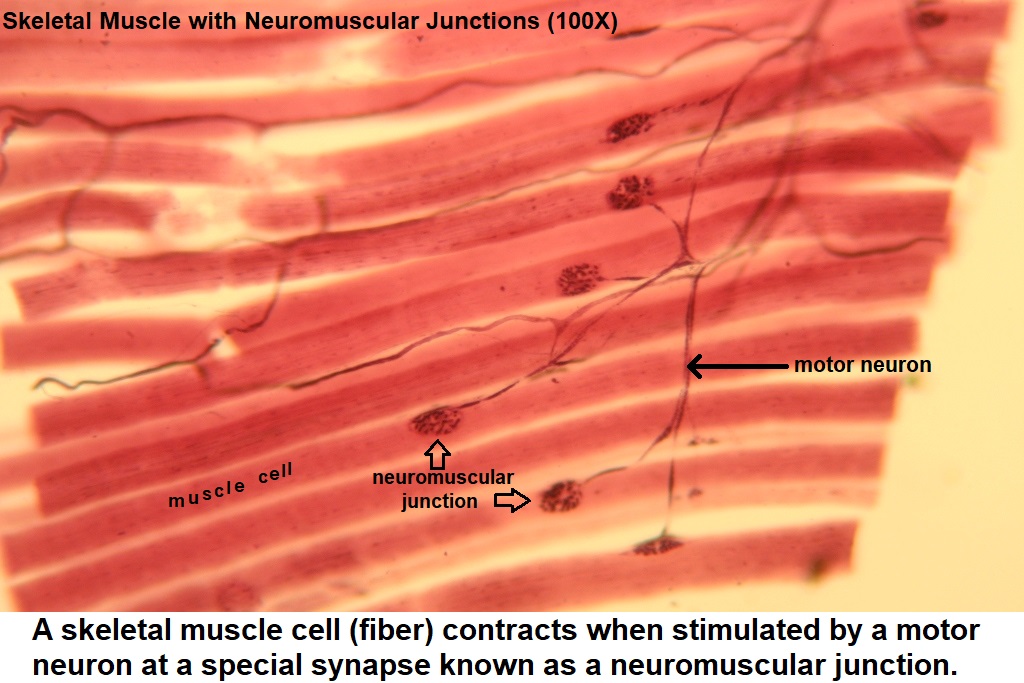The image is a rectangular diagram, approximately 5 to 6 inches wide and 4 inches high, often found in scientific papers or textbooks. It features a detailed illustration of skeletal muscle and neuromuscular junctions. The background is a light yellowish-tan, with horizontal red-striped muscle cells that include red tendrils and small red dots with yellow highlights. In the top-left corner, bold black print reads "Skeletal Muscle with Neuromuscular Junctions (1000x)." The middle-right side of the image labels the red tendrils as "motor neuron" with arrows, and further to the left, two more arrows indicate the "neuromuscular junction." The muscle cells are detailed with horizontal slats and red dots. Along the bottom of the image, black bold text on a white background states, "A skeletal muscle cell (fiber) contracts when stimulated by a motor neuron at a special synapse known as the neuromuscular junction."